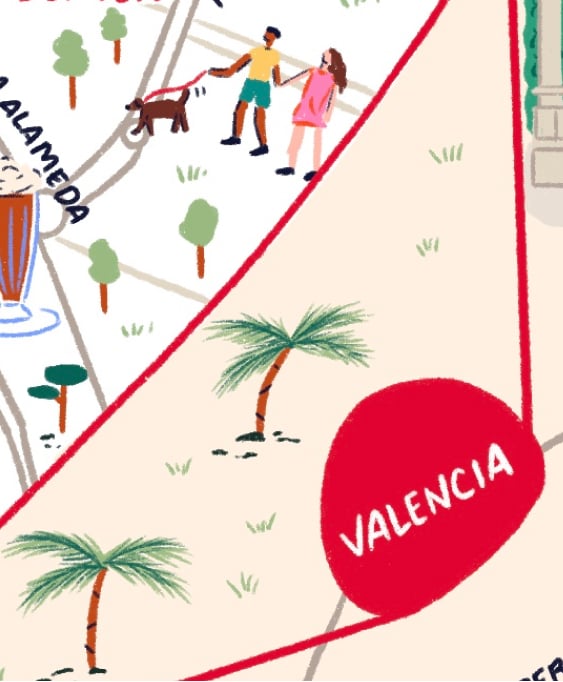This image is a vertically-oriented poster that possibly depicts a map-like illustration. The design is divided diagonally from the bottom left to the top right. The lower right section, which covers about two-thirds of the image, features a light brown background with a texture resembling sand. In this section, the word "Valencia" is prominently displayed in white capital letters, encased within a rough, red, oblong, non-symmetrical circle. Extending from this circle are two red lines moving either upwards or to the left.

In the upper left portion of the image, there are color drawings of a man and a woman walking a brown dog. The man, who appears to be Black, is wearing a yellow or white t-shirt and teal shorts, with black shoes. The woman, who seems to be Caucasian, is dressed in a pink dress with black shoes and has long brown hair. The dog they are walking is on a red leash. This part of the image also contains beige or brown lines indicating roadways, flanked by three or four trees, including palm trees. Additionally, the word "Alameda" is visible in the background here, along with a glass that looks like it contains a root beer float or beer, positioned at the left side of the upper section.

Overall, the illustration blends elements of a scenic walk with a hint of cartographic representation, emphasizing the places named "Valencia" and "Alameda" along with the relaxed ambiance of people strolling with their dog amidst palm trees.